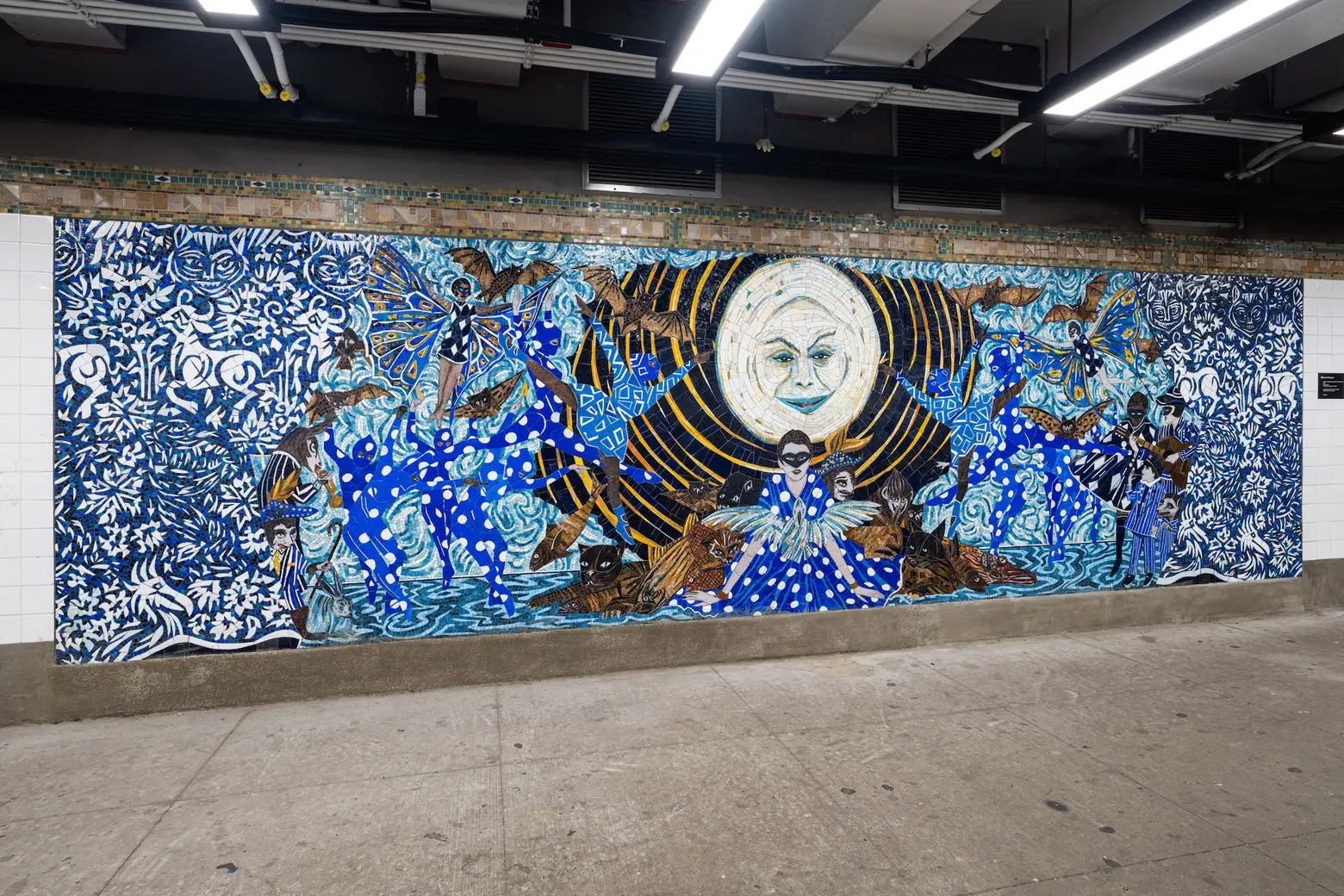This photograph features a vibrant and fantastical mural on a wall in an urban setting, possibly in a public place like a subway station or school hallway. The floor in front of the mural is paved with large concrete slabs, and the ceiling is composed of different metals with beams of white light. The mural, which measures less than 20 feet in length and about a story in height, is predominantly blue with various shades ranging from light to dark, accented with white and gold.

At the heart of the mural is a circular object resembling the moon, complete with a face that appears to be gazing down at a person sitting on the ground. The person, who might be a child in a blue dress with white polka dots, is surrounded by a captivating array of flying creatures such as butterflies, fairies, and bats. The mural also depicts whimsical figures including mountain goats, lions, bulls, and perhaps a rooster, all set against a backdrop of colorful dots, shapes, and intricate patterns. The entire scene blends abstract elements with surreal imagery, creating a mesmerizing and dreamlike atmosphere.